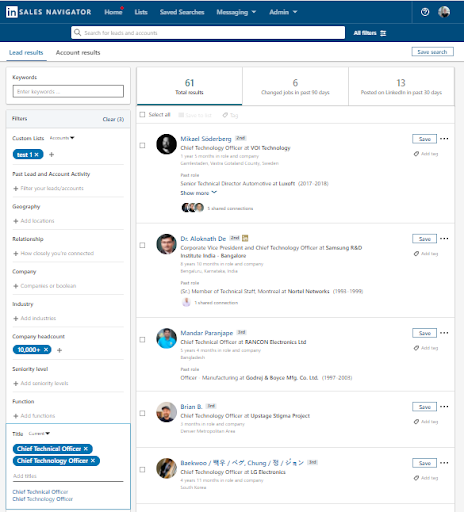This image is a screenshot from Sales Navigator. In the upper left corner, there is a white rectangular block containing the word "End." Moving right, the Sales Navigator logo is positioned in a blue bar that spans the width of the image from left to right. 

On this blue bar, to the right of the Sales Navigator logo, is the menu. The menu items listed are: "Home," "Lists," "Saved Searches," "Messaging," and "Admin." 

Directly below this menu, and still within the blue bar, there is a search bar centered in the middle. 

Below the blue bar is the main window displaying lead results. The upper left portion of this white main window contains two tabs: "Lead Results" and "Account Research Results," with "Lead Results" currently selected. 

To the left of the main window, there is a vertical menu. On the right-hand side, there are three tabs at the top resembling boxes. The selected tab displays "61 Total Results." 

The main content area shows five individual objects listed as lead results.